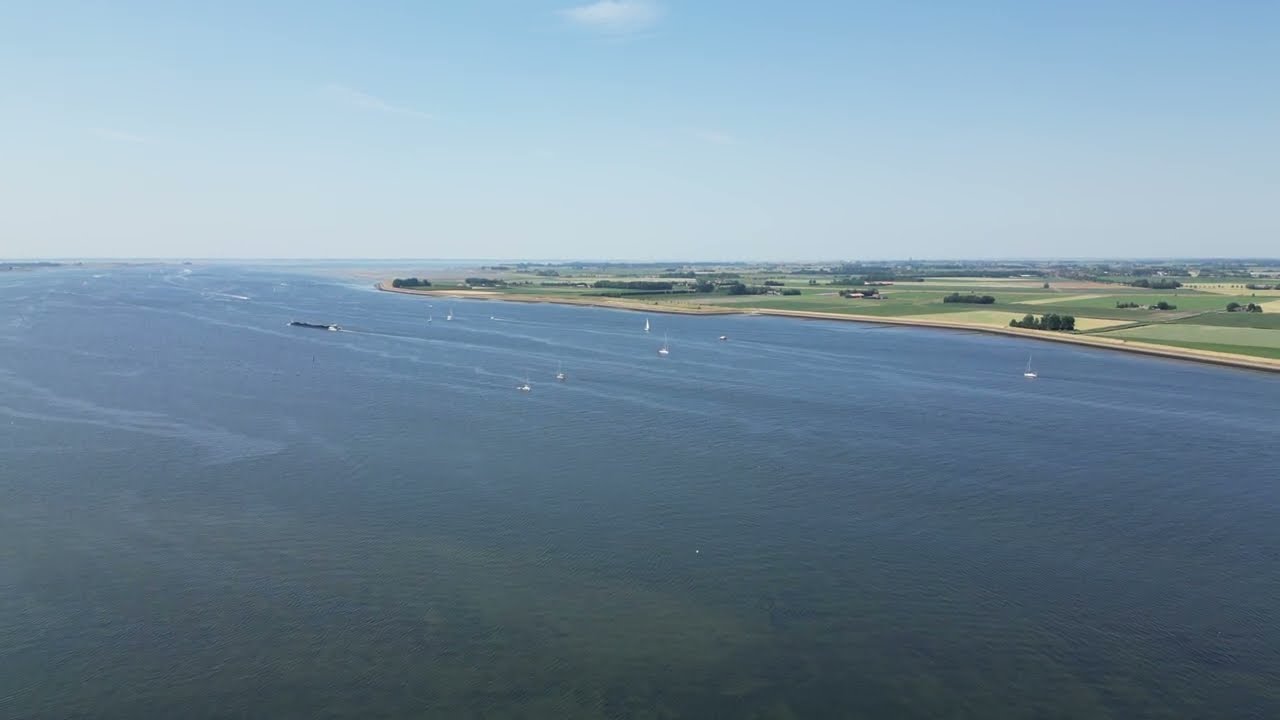This aerial image captures a serene and expansive body of water, predominantly a dark blue with occasional streaks suggesting reflections from various structures, creating a calm yet dynamic scene. Scattered across the water are multiple white and gray sailboats, adding a touch of activity to the tranquility. A noticeable feature on the left side near the center is a black line-like object bordered in white, likely a barge. The horizon lines the upper portion of the image, where the sky transitions from a clear, faintly hazy blue at the top to a lighter, almost grayish-blue near the horizon.

In the upper right section, the shoreline presents a richly variegated landscape. Here, one observes a mix of dark green, light green, and yellow patches, indicative of farmland with interspersed green vegetation, bushes, and trees. The land displays a blend of textures and colors – from the dark brown shoreline to lighter sandy areas further inland. Some of these patches likely pertain to grassy fields, crops, or gardening areas. Among these farmlands, some gray structures resembling buildings suggest a potentially commercial real estate area, interspersed with smaller clusters in the distance.

At the very top center of the image, a wispy white cloud graces the otherwise mostly clear sky, contributing to the peaceful yet detailed tableau captured from the aerial perspective.